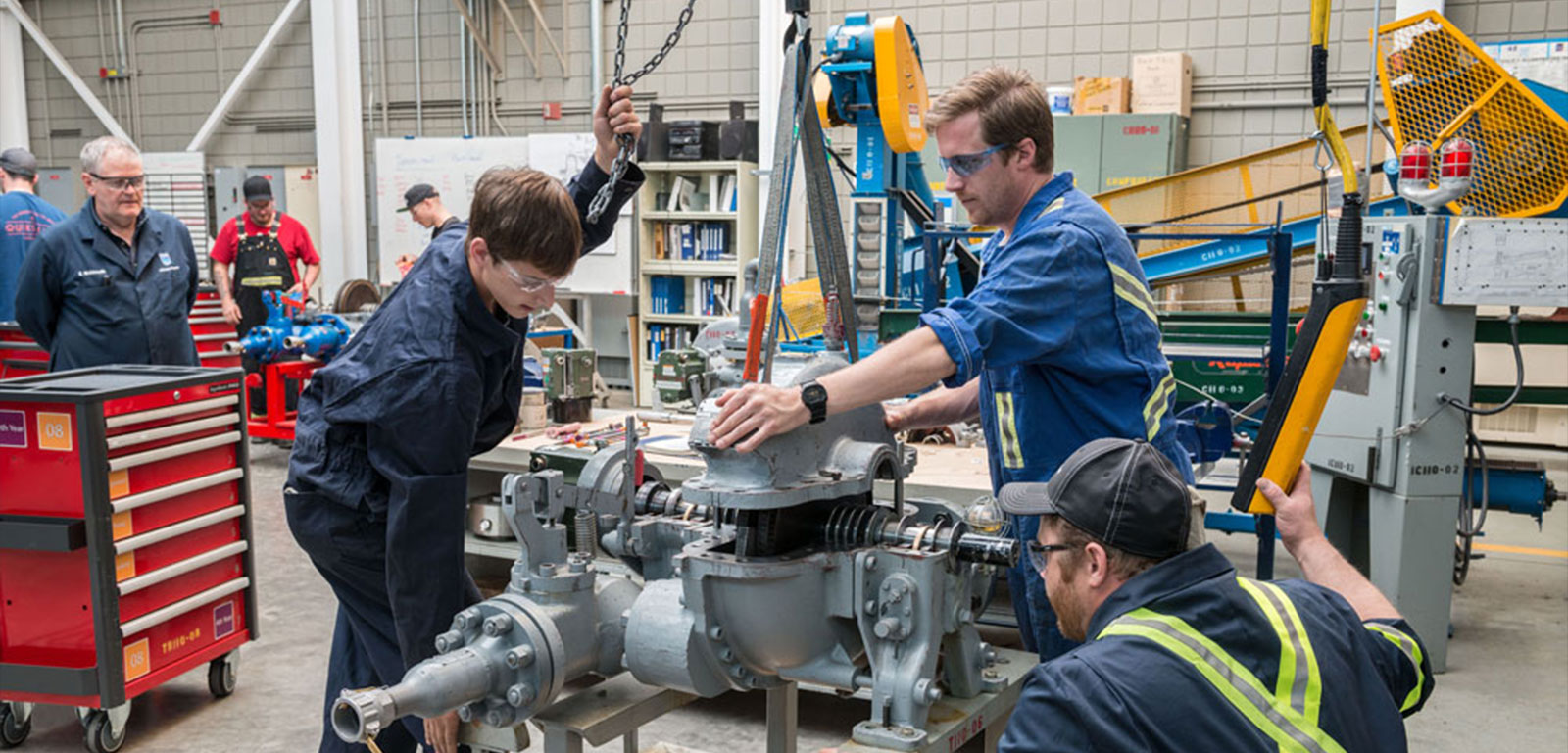The image captures the interior of a factory or mechanical workshop, bustling with activity and various machinery. In the foreground, three men in blue coverall work uniforms, all wearing goggles, are intensely focused on a large prototype metal machine. The man on the left, kneeling, appears to be handling a yellow component, possibly attached to a chain from the ceiling. The central figure stands with his hands on the machine, while the younger man to the right holds a chain above his head, steadying the bottom part of the machine. To the far left, a red tool case is visible, and an older man in coveralls observes the trio’s progress. The background reveals additional workers engaged in their tasks amidst different types of machinery. A bookshelf housing numerous manuals is also visible, indicating a highly technical and instructional environment. The scene is energetic and detailed, filled with the organized clamor typical of a professional engineering setting.